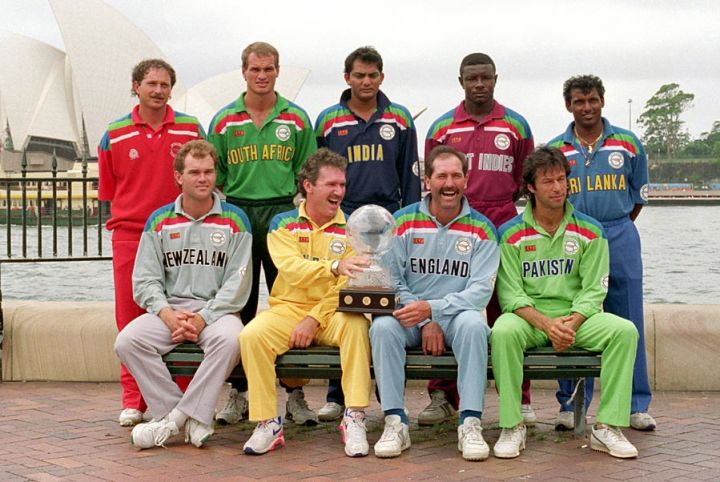The image captures a diverse group of nine men posed for a photograph, holding what appears to be a World Cup trophy for a sporting event. The group consists of individuals from various racial backgrounds, including White, European, Indian, and African-American, with their hair ranging from dark brown to almost black.

In the front row, four men are seated. The man on the far left is dressed in a gray suit representing New Zealand. Next to him, a man wearing a yellow outfit holds the translucent globe trophy on a base, partially obscuring his attire. The third individual from the left sports a pale blue outfit signifying England, while the man on the far right dons a medium neon green attire symbolizing Pakistan.

The back row features five standing men in an array of track suits, each denoting their respective countries. From left to right: the first man wears a red outfit, though his country remains unidentified. The second man is in a green shirt emblazoned with "South Africa." Next, a man in a dark blue track suit represents India. To his right, a man dressed in red signifies West Indies. The final man on the far right is clad in a medium blue outfit representing Sri Lanka.

Their varied attire and the prominent trophy suggest a celebration of international sportsmanship and camaraderie, possibly at a World Cup event.